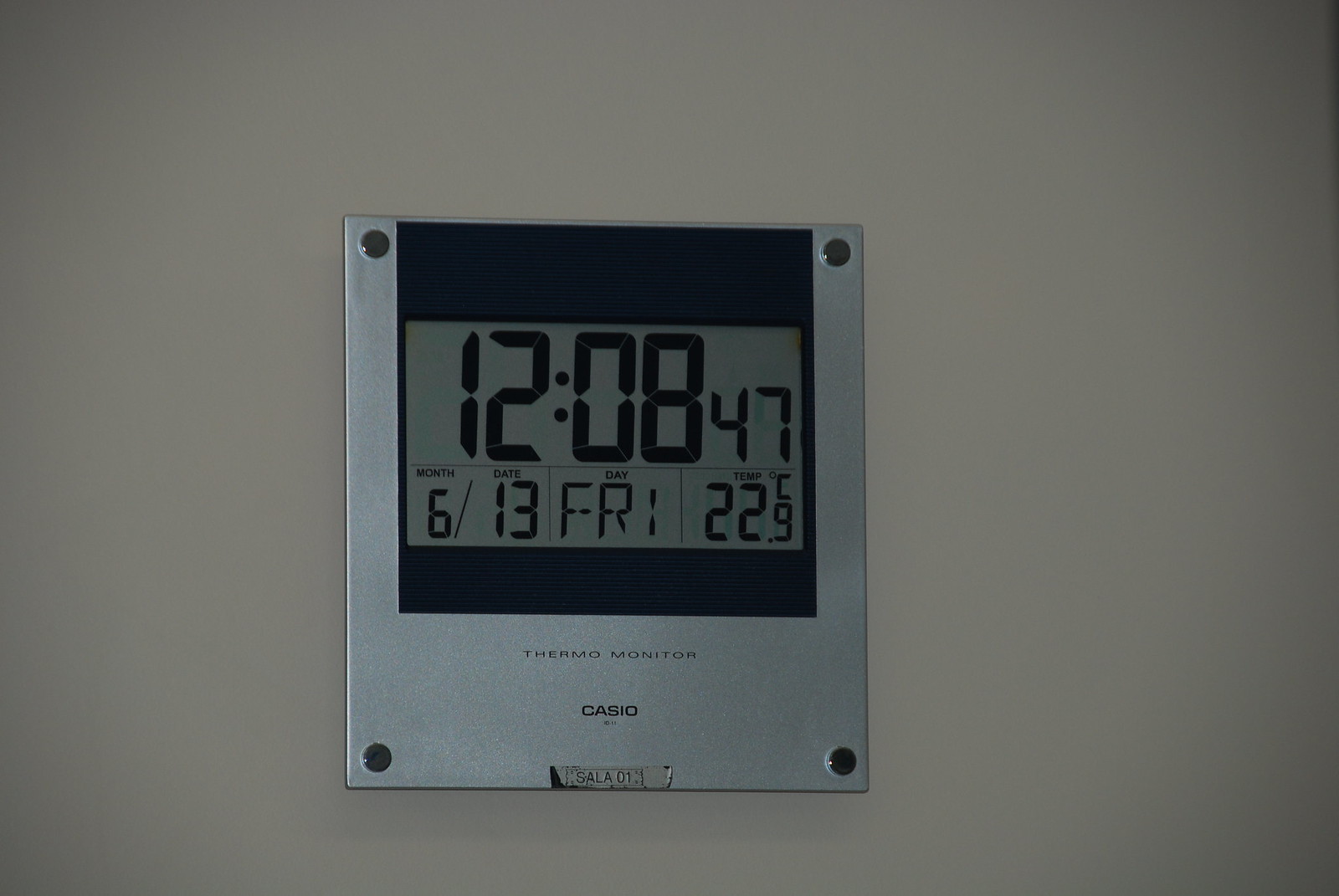This image depicts a silver digital thermal monitor mounted on a wall. The screen displays the current time as 12:08:47, with the date specified at the bottom left as Friday, June 13th. The temperature reading is indicated as 22.9 degrees Celsius. The bottom of the monitor features the words "Turbo Monitor" in a very thin font. Above this, there is a distinctive "Casio" logo, and beneath it, the model designation "SA LA 01" is visible. Each corner of the monitor's plate has a black circle, adding a touch of symmetry and design contrast to the otherwise sleek, metallic finish.